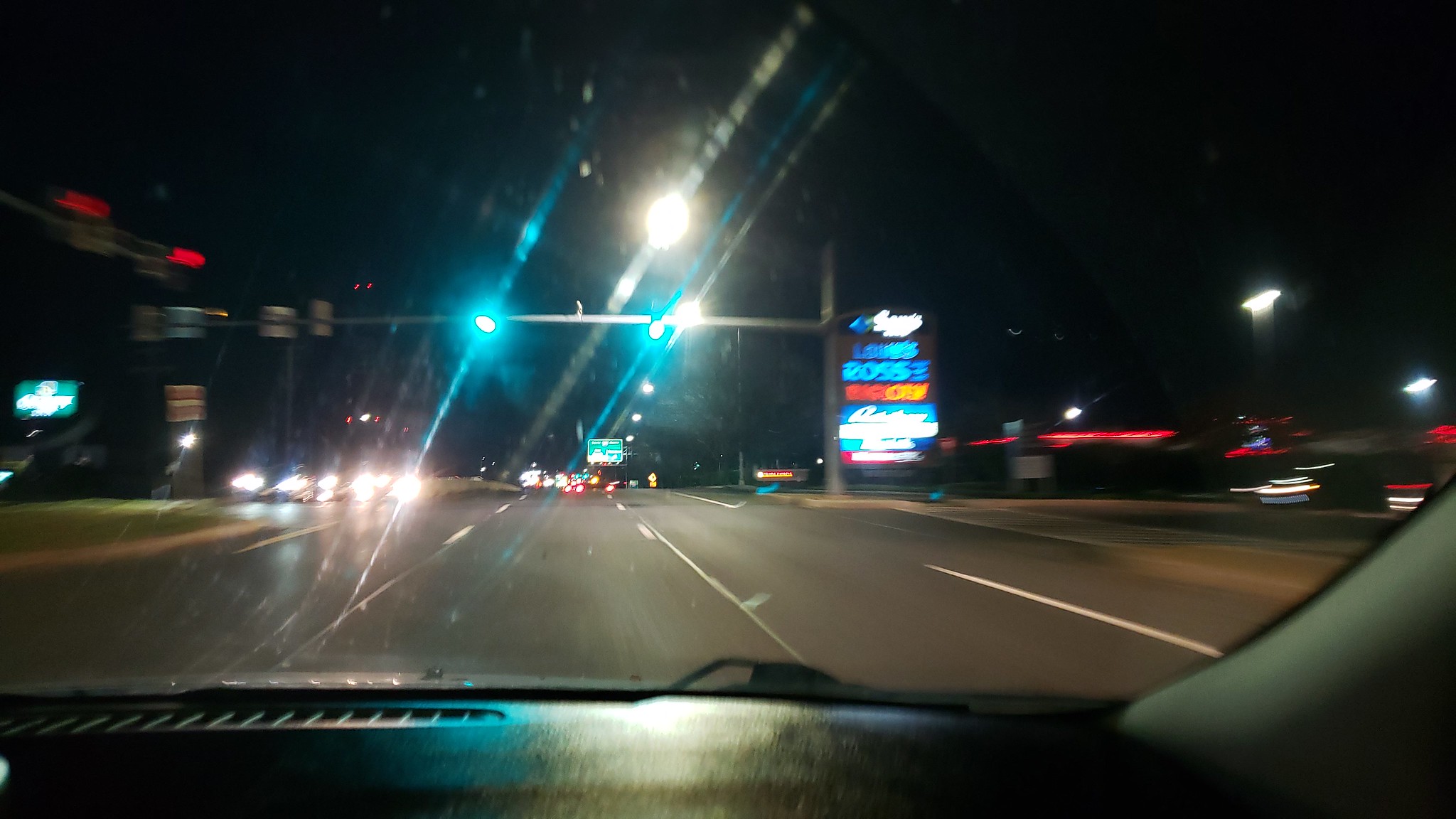A scene viewed from inside a vehicle showcases a reflective plastic dashboard, revealing a detailed interior. On the right side of the dashboard, a white glass object is visible, catching the light and producing a noticeable glare. Distant lights flicker ahead, creating a captivating play of illumination in the dark setting. The sky in the background is a deep black, providing a stark contrast. To the left, faint traces of red hint at previous illuminations or reflections. On the right side, the view extends to grass, with additional elements contributing to a compelling and multifaceted landscape punctuated by various lights.